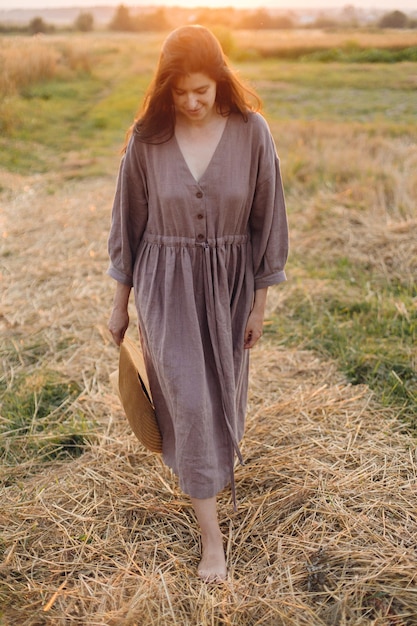The colour portrait photograph depicts a lone woman standing in the center of a grassy field strewn with straw and hay, which is deep and yellowed. She is barefoot and looking down at her feet or the ground, obscuring her eyes from view. She is dressed in an old and tired-looking, baggy, brown one-piece dress with three buttons buttoning a deeply cut V-neck. The dress features slightly turned-up cuffs and an elastic cinching at the waist. Her long hair, lightened by the sunlight streaming in from behind, falls over her shoulders with darker shades at the sides. In her right hand, she carries an object that appears beige and is possibly a wooden pot. The background is composed of uneven grass and yellow fields, with some shrubs and trees visible on the distant horizon line, and possibly the sky, although it is hard to discern. The setting sun illuminates the scene, giving a warm glow to the back of her head.